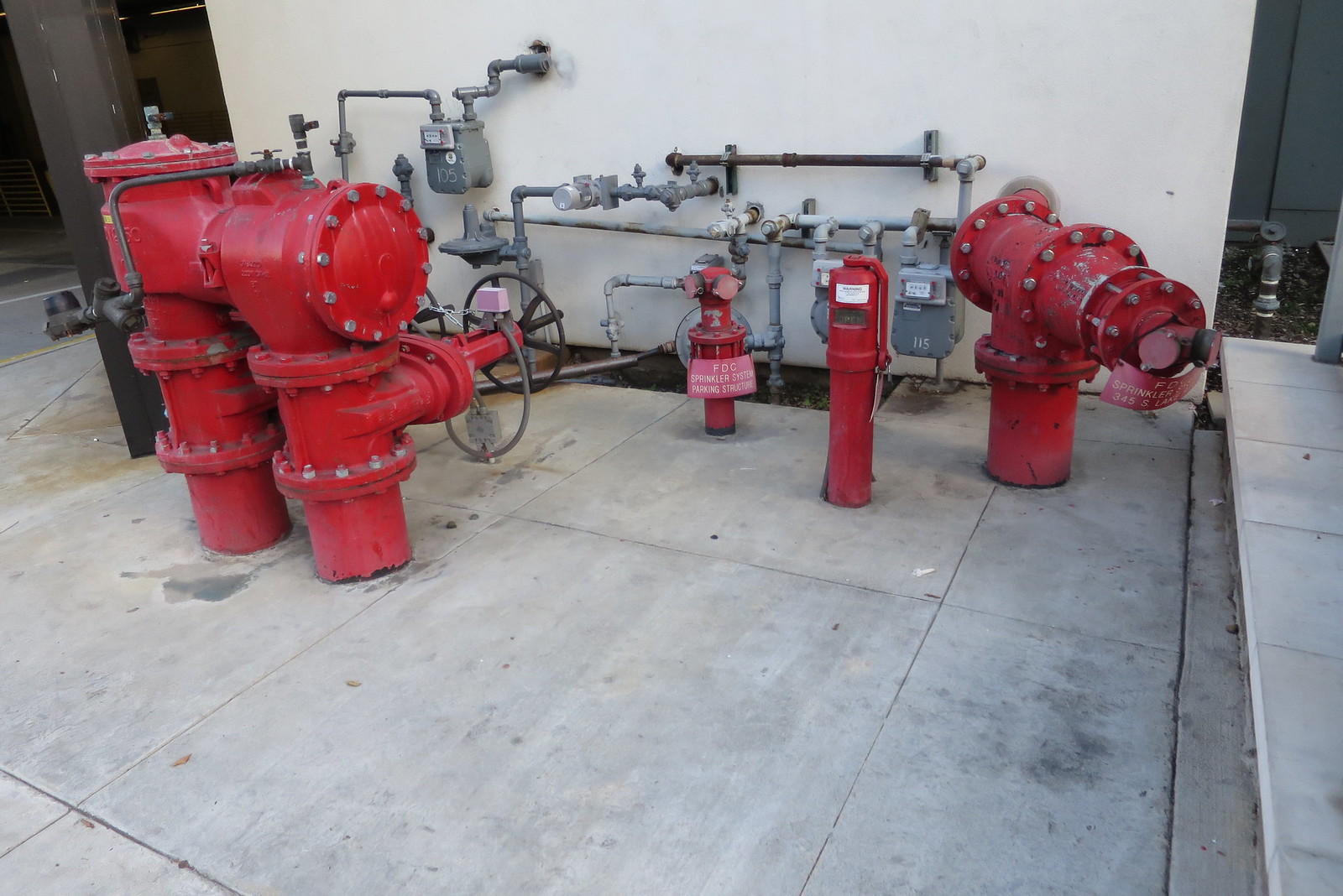This is a detailed color photograph of an industrial setting, likely part of a factory or fire control system. Prominently featured are bright, vibrant red pipes connected to substantial silver metal pipes that extend from a white, stucco wall. Multiple handles and large bolts are visible on these pipes, indicating different control points and secure fittings. The arrangement includes a red valve tower and what appear to be fire hydrants. A sign marked "FDC" suggests these may be part of a fire department connection system. The floor consists of concrete slabs, displaying some dark patches and stains, indicative of heavy usage and wear. Additionally, there is a wheel with an attached hose, and three meters mounted on the wall, further contributing to the suggestion that this setup is integral to a building's utility or fire safety infrastructure. The scene is devoid of people, focusing solely on the complex piping system.